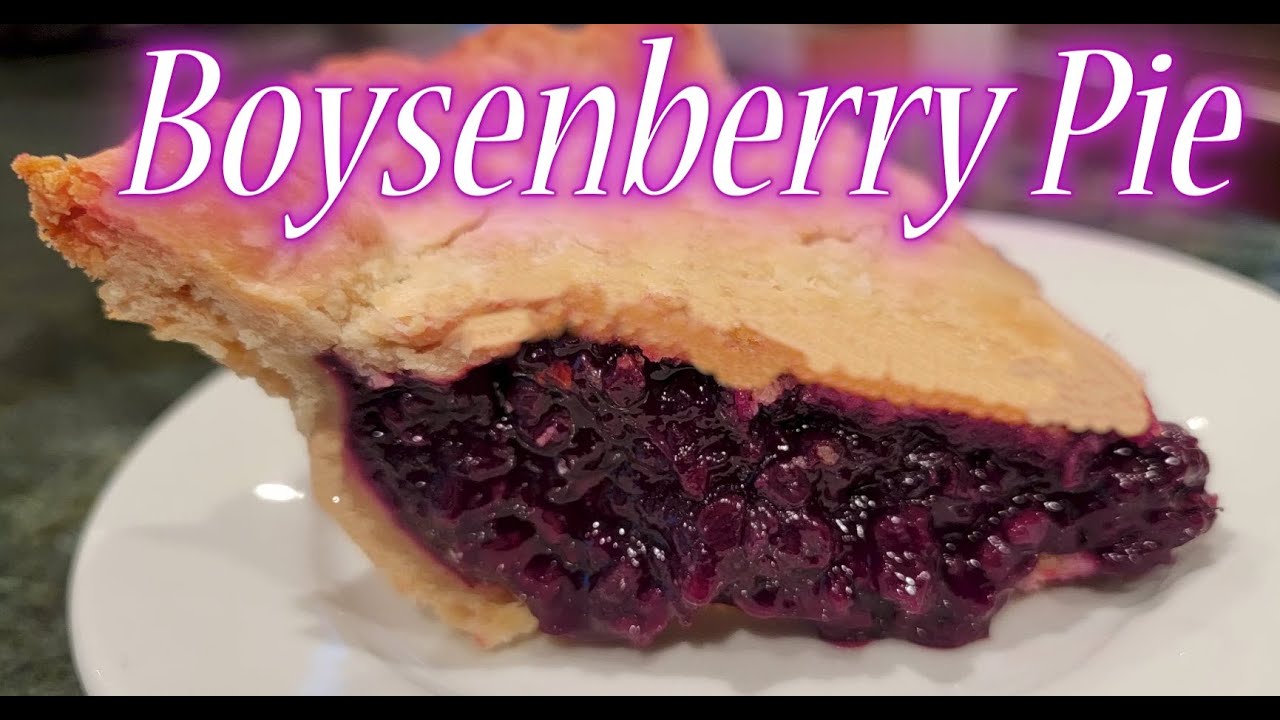In the image, an appetizing slice of boysenberry pie takes center stage, sitting on a pristine white ceramic plate that rests on a neutral gray table, possibly granite. The pie's filling is a luscious, moist blend of dark purple and red boysenberries, surrounded by a beautifully flaky crust. The crust is golden brown, with the edges appearing darker and more well-cooked. The background of the image is intentionally blurred, keeping the viewer's focus on the delectable dessert. Adding to the visual appeal, the words "boysenberry pie" are prominently displayed at the top in a glowing white text with a neon purple edge, suggesting a professional advertisement, perhaps for a restaurant or patisserie. The image conveys the pie's deliciousness through its vivid colors and inviting textures.